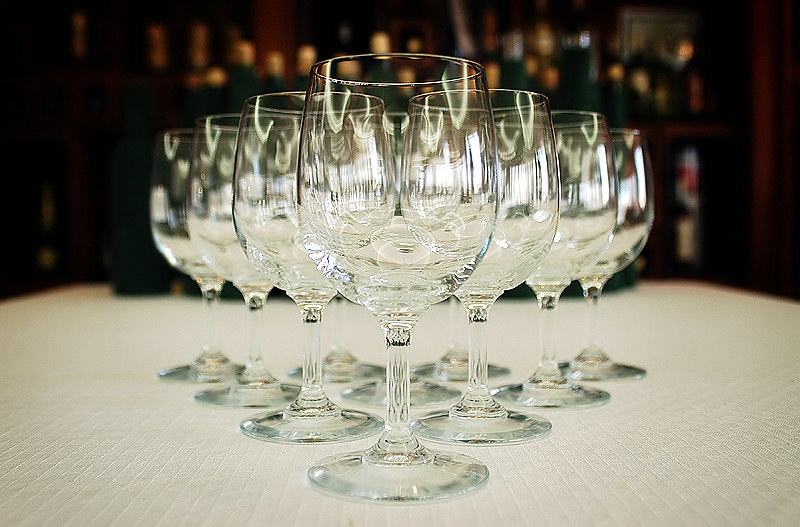This professionally taken photograph captures the elegant interior of a fancy restaurant. The focus of the image is a clear wine glass positioned at the center of a white tablecloth, which features a sophisticated texture with square patterns. This tablecloth spans from the left center to the right center, extending downwards towards the bottom edges of the frame.

Arranged in a pyramid formation starting from the front, there is a single wine glass in sharp focus followed by two, three, and finally, four glasses consecutively positioned behind it. Each glass is meticulously crafted with detailed stems that slightly curve out, and as they recede into the background, they progressively blur into the distance. These sparkling clean glasses give a sense of depth through their alignment, with reflections and openings adding to the intricate visual layering.

In the blurred background, the ambiance is set with shades of dark brown, black, and beige, interspersed with what appears to be the tops of various bottles in yellow-gold hues, suggesting a bar atmosphere. The frontmost wine glass almost fills the entire height of the frame, emphasizing the meticulous detailing of the stem and base, while the progressively blurrier rows enhance the perspective and elegance of the arrangement.